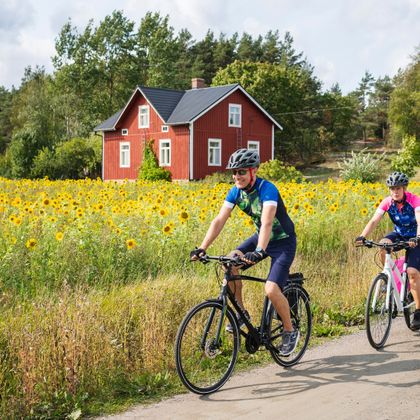This photograph captures a picturesque summer scene of a couple riding hybrid bicycles on a dirt road through the countryside. The man, in a blue shirt with green accents, blue shorts, and blue tennis shoes, leads the way on his black bike, sporting sunglasses and a black and green helmet. The woman follows closely behind, dressed in a pink and blue shirt with black shorts, her white bike complementing her outfit. Both riders wear matching black and green helmets, highlighting their coordinated attire for the outdoor adventure.

To their left stretches a vast field densely packed with vibrant sunflowers, while grassy patches line the edges of the dirt road they traverse. In the distance, a quaint red house with white-trimmed windows and a black roof, complete with a chimney, stands amidst tall, green trees, suggesting early summer. The clouds dotting the sky above add to the serene rural backdrop. This idyllic setting, potentially reminiscent of Kansas, frames a charming moment of shared exploration and companionship.